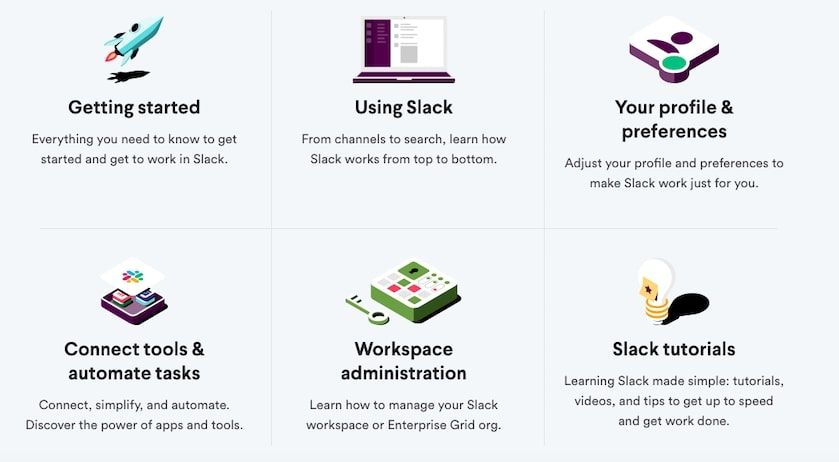The image features a light gray colored box divided into six distinct sections, each providing detailed information about navigating Slack.

**Top Left Section**:
- **Illustration**: A rocket ship icon
- **Bold Text**: "Getting Started"
- **Description**: "Everything you need to know to get started and get to work in Slack."

**Middle Left Section**:
- **Illustration**: An icon representing a laptop screen
- **Bold Text**: "Using Slack"
- **Description**: "From channels to search, learn how Slack works from top to bottom."

**Top Right Section**:
- **Illustration**: A generic profile picture with a green status circle
- **Bold Text**: "Your Profile and Preferences"
- **Description**: "Adjust your profile and preferences to make Slack work just for you."

**Middle Right Section**:
- **Illustration**: An unspecified key and a device with numerous buttons
- **Bold Text**: "Advanced Features"

**Bottom Left Section**:
- **Illustration**: An icon representing tools
- **Bold Text**: "Connect Tools and Automate Tasks"
- **Description**: "Connect, simplify, and automate. Discover the power of apps and tools."